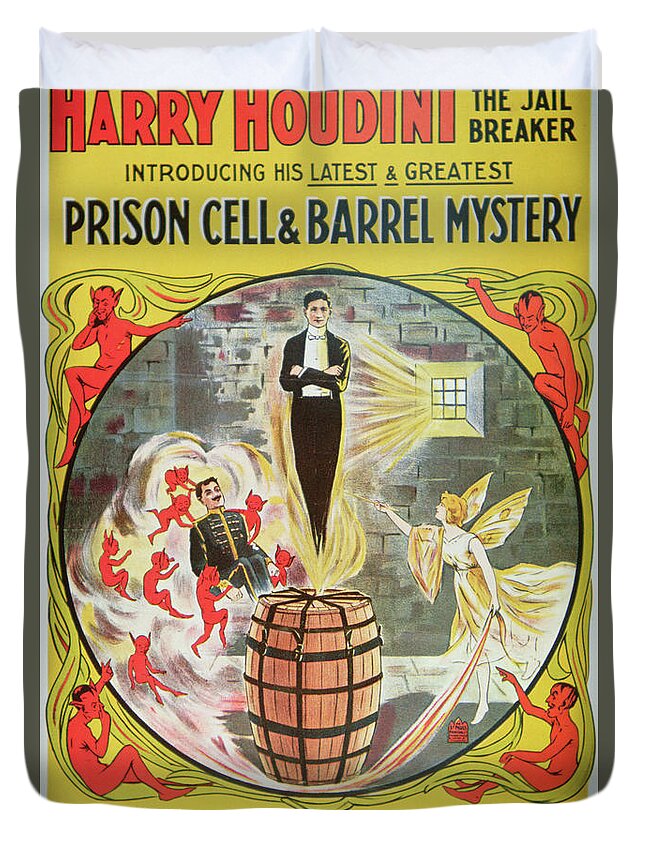This is a vintage, professionally drawn poster from the 1910s or 1920s for Harry Houdini, showcasing his "latest and greatest prison cell and barrel mystery." At the top of the poster, the text "Harry Houdini the Jailbreaker" is prominently displayed in red, with additional information in black text. Dominating the center is a circular illustration where Houdini, depicted in a black suit with black hair, hovers above a barrel wrapped in many straps. Yellow lines resembling flames emanate from the barrel, adding a dramatic effect. An angel with wings reaches out towards Houdini from the right, while to his left, a figure in a military uniform is surrounded by swirls and eight small red devils. These devils, red and naked with pointed ears and masculine features, also appear at each corner outside the circle, either pointing at or observing Houdini. The background suggests a prison cell, complete with gray cinder blocks and a small window featuring nine small squares, through which light streams in, emphasizing the dungeon-like atmosphere of the scene.